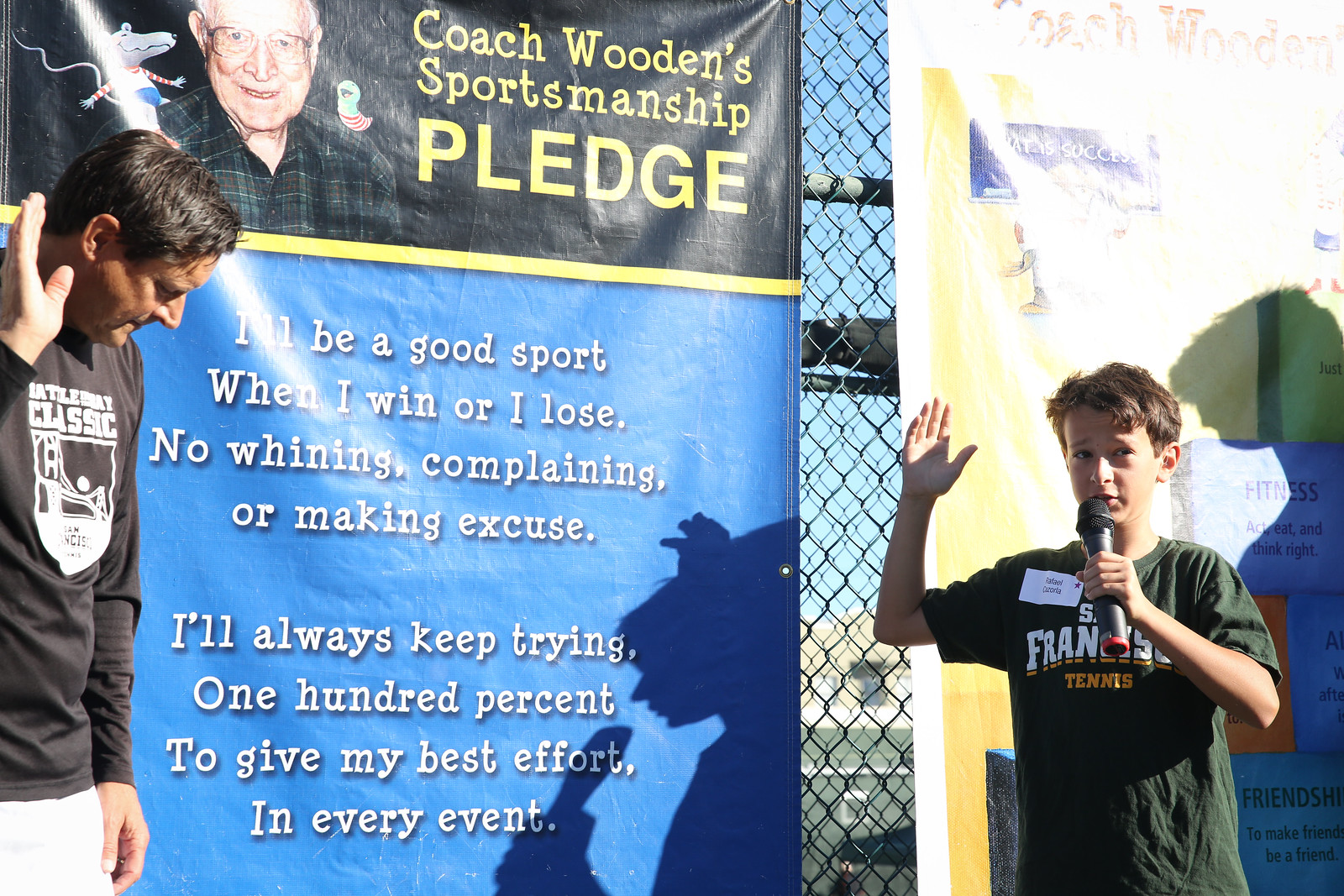In this vibrant outdoor photograph, a young boy, approximately 10 years old, is captured mid-speech, holding a microphone in his left hand. He is energetically addressing an audience while wearing a short-sleeved army green t-shirt with white lettering that reads "San Francisco Tennis." Bathed in the bright sunlight, his shadow is prominently cast behind him. To his left stands a man, possibly his coach or father, partially cut off in the frame. The man, with short brown hair, is dressed in a long black-sleeved shirt and white pants or shorts, and his right hand is also raised, suggesting he might be leading or participating in a pledge. Behind them, a chain-link fence displays two banners. One of the banners features "Coach Wooden's Sportsmanship Pledge," which includes a commitment to being a good sport, not whining or making excuses, and always giving 100% effort. The scene is set in a daytime outdoor venue, likely at a sporting event, capturing a moment of earnest engagement and youthful enthusiasm. Various colors like blue, yellow, black, white, silver, beige, and light blue are evident in the surroundings, adding to the lively atmosphere of the photograph.